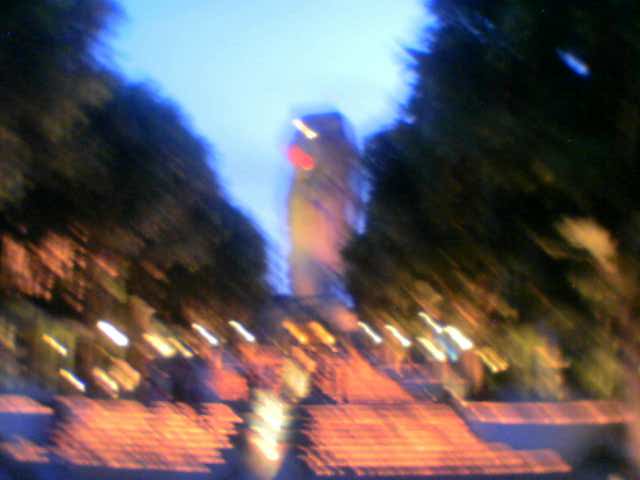The image is very blurry, likely due to motion blur from the photographer or the environment. At the center, there is a large statue or structure with a light green backdrop, possibly the sky, which is a bright, light blue suggesting either sunrise or sunset. The bottom portion of the photo features stone stairs leading up toward the central statue. Along the sides of the stairs, there are horizontal strings of lights in a mix of white and orangish-yellow hues. Flanking the stairs, large trees with dark green leaves and brownish branches create a leafy frame. Though the details are obscured, no text or figures are visible. The colors around the statue and stairs include light pink, blue, yellow, and white patches, adding to the overall ethereal, blurred ambiance.